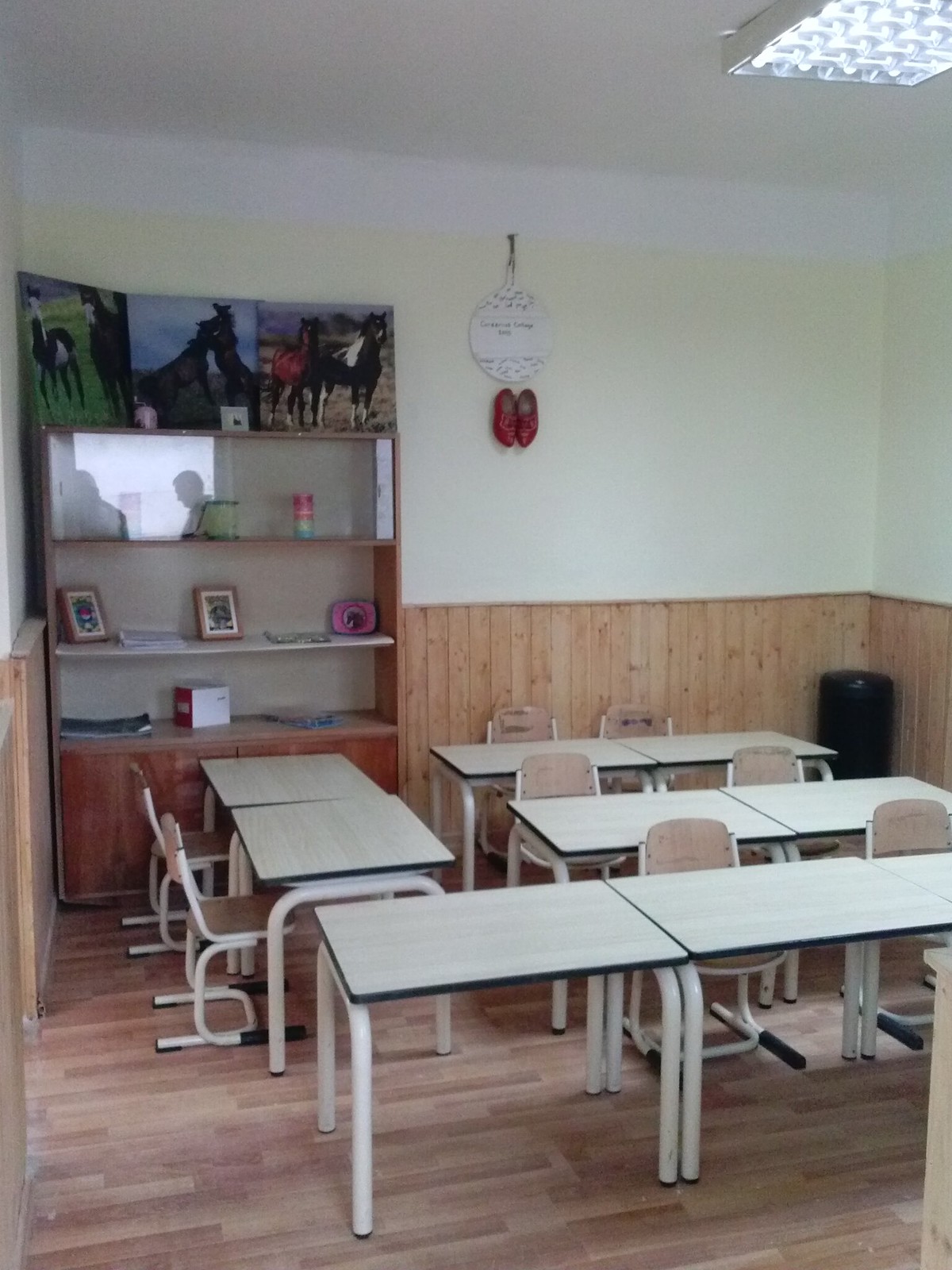The photograph shows the interior of a small classroom. The ceiling is white, with rectangular lights visible at the cut-off top right-hand corner. The walls are light cream-colored with wooden paneling halfway up, separated by a small wooden trim. The floor is covered in brown wood or laminate tiles. There are eight off-white desks with black outlines and white legs arranged in rows, mostly in pairs, although the front row appears to have three desks. The grayish-back chairs have white metal legs matching the desks. On the left side of the room, there's a large wooden cabinet. The top shelf has a glass front showcasing some ornaments, while the middle shelves are open and display pictures, frames, and cardboard boxes. The lower section of the cabinet features additional cupboards.